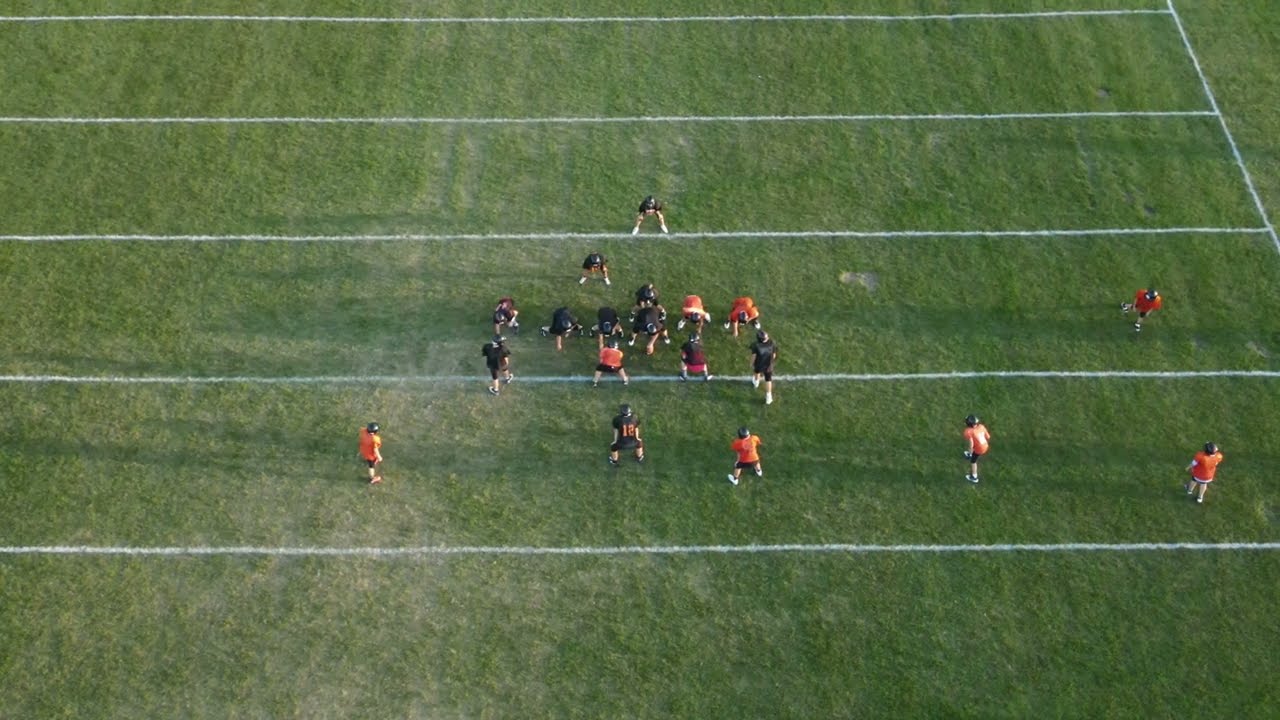This aerial photograph captures a daytime scene of a peewee football game on a green grass field, partially worn to dirt from frequent play. Two teams, children aged approximately 7 to 10 years old, are distinguishable by their uniforms: one team wearing orange jerseys and black shorts, and the other in black jerseys—with some variations where orange numbers are visible. The players are lined up in offensive and defensive formations, with white yardage lines painted across the field clearly marking distances. Notably, the left side of the field is brightly lit with sunlight, while the right side appears slightly shaded, casting a yellowish hue on the more illuminated parts. The scene suggests action is about to commence, with wide receivers and other players in position, all equipped with helmets. There are no spectators on the sidelines, indicating it could either be a game or practice session.